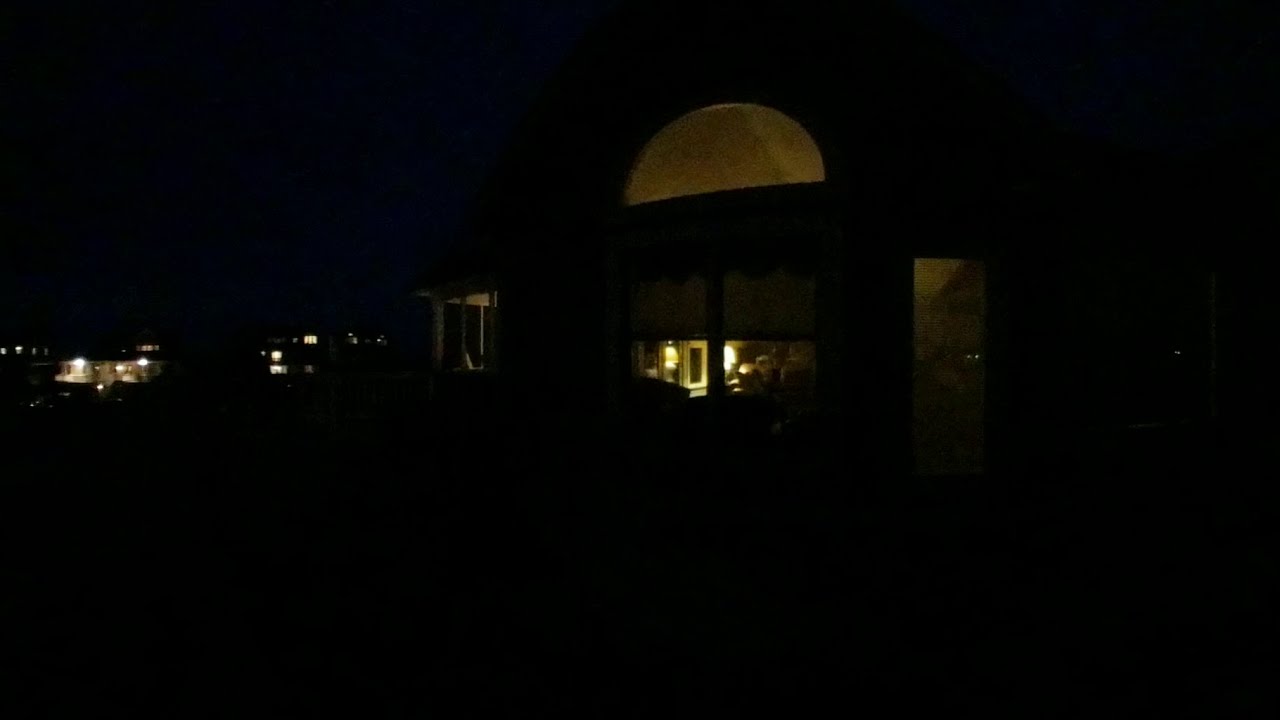The photograph depicts a nighttime scene dominated by darkness, with only a few sources of light providing subtle illumination. Predominantly black, the image captures a large house situated somewhat to the left. This house features a porch with its light on, highlighting the facade facing slightly to the left. Additionally, the house has two prominent big rectangular windows and a half-circle window above a set of double doors, all glowing due to the interior lights. No people are visible inside, but the lit glass door and windows reveal a warmly lit room, creating a cozy atmosphere. In the background, there appears to be an upscale neighborhood, as several other large houses are barely discernible but for the lights radiating from their windows. Apart from the household lights, the scene is largely devoid of illumination, with no visible stars or moon to break the darkness.